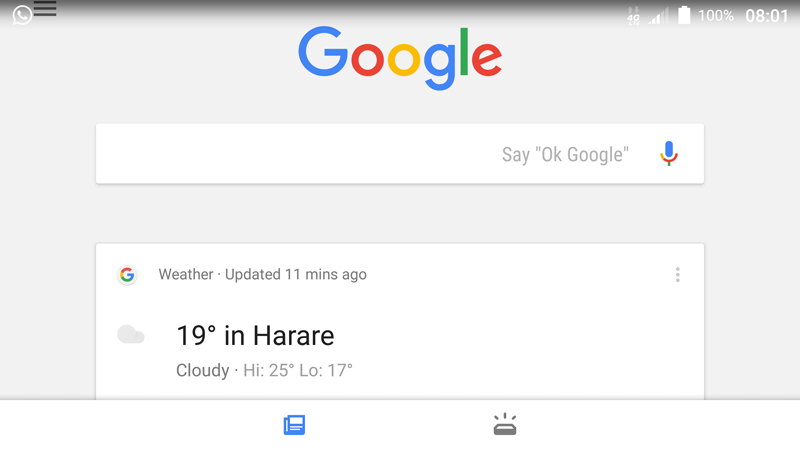This image captures a Google search screen in detail. The top section of the screen features a status bar, which includes a circle icon with a phone on the left, followed by a three-line menu icon. To the far right, the status bar displays "4G," indicating the network connection with three bars of signal strength. Adjacent to this, the battery icon shows a full charge at 100%, and the current time is displayed as 8:01.

Prominently centered on the screen is the Google logo, stylized with the letters in specific colors: the first "G" in blue, the first "O" in red, the second "O" in yellow, the second "G" in blue, the "L" in green, and the "E" in red. Below the logo is an empty search bar containing the text "Say OK Google" alongside a microphone icon, indicating voice search functionality.

Directly beneath the search bar, there is a weather update displayed in a square format. The weather update indicates it was refreshed 11 minutes ago and features a "G" on the left, signifying that the information is sourced from Google. The weather update provides details for Harare, noting that it is currently 19 degrees Celsius and cloudy, with a high of 25 degrees and a low of 17 degrees.

The background of the screen surrounding the weather update and search bar is an off-white or very light gray color, creating a clean and minimalistic appearance. Overall, this is a crisp and detailed snapshot of the Google search interface.